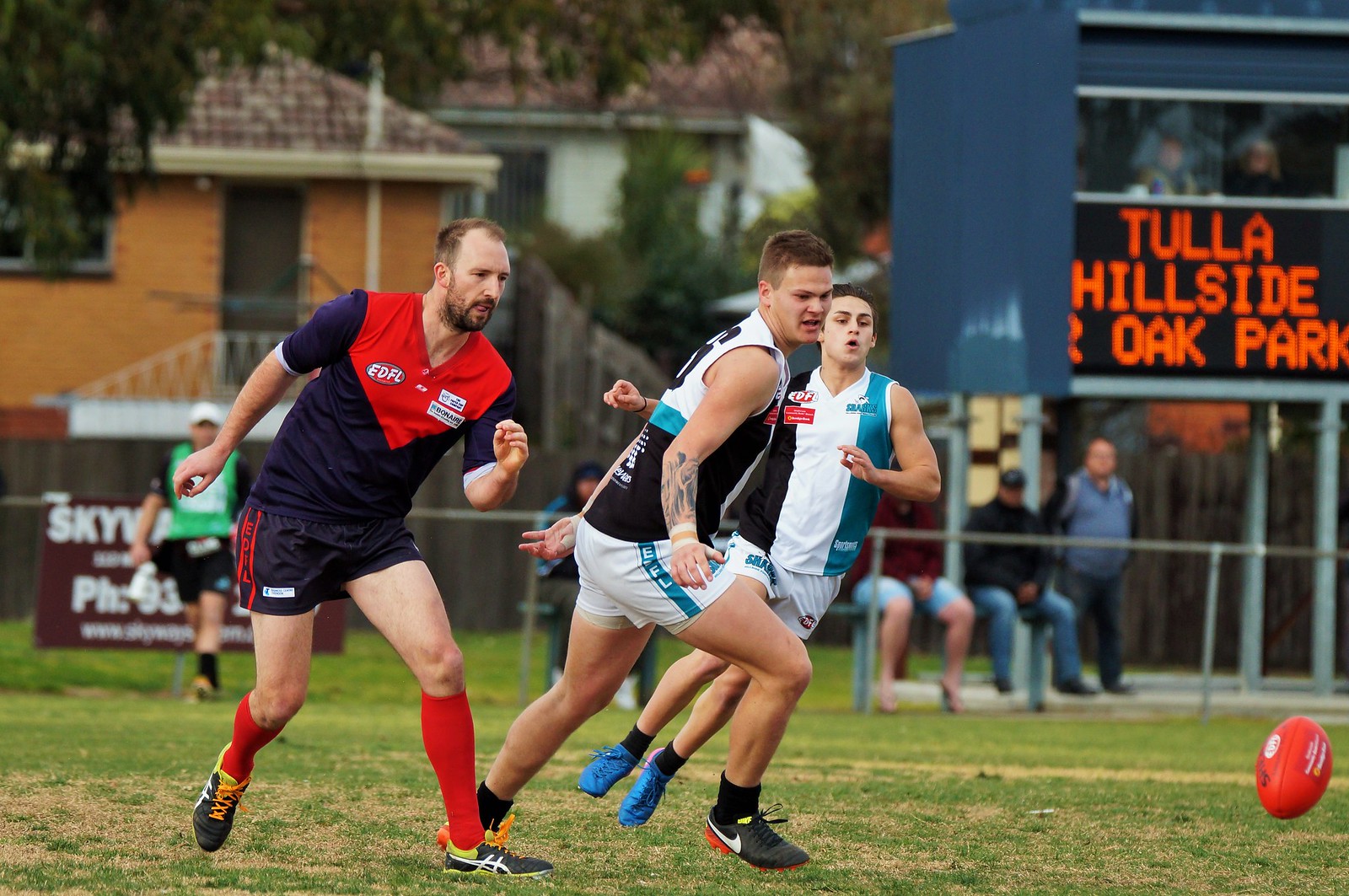The image depicts a lively football game with three young male players sprinting across a lush green field towards a brown leather football that is situated in the bottom right corner. The players are distinguished by their uniforms: two are clad in white, black, and teal sleeveless jerseys with white shorts, while the third player on the left wears a dark blue jersey with red shoulders, red high socks, and dark blue shorts featuring a red stripe down the middle. The scene is complemented by the presence of a referee in the background, dressed in a green pinny and black shorts.

Framing the action, a chain-link fence runs along the back, adorned with a banner or advertisement. Behind this fence, four spectators sit on a bench, watching the game intently. Off to the left, an official can be seen strolling on the field. In the upper right section of the image, a black digital scoreboard with red letters displays "Tullow Hillside Oak Park," positioned near what appears to be an announcers' area with additional seated individuals.

Beyond the immediate field of play, the background reveals a quaint neighborhood with some yellow and white houses partially obscured by trees, further enriching the scene's detailed setting.